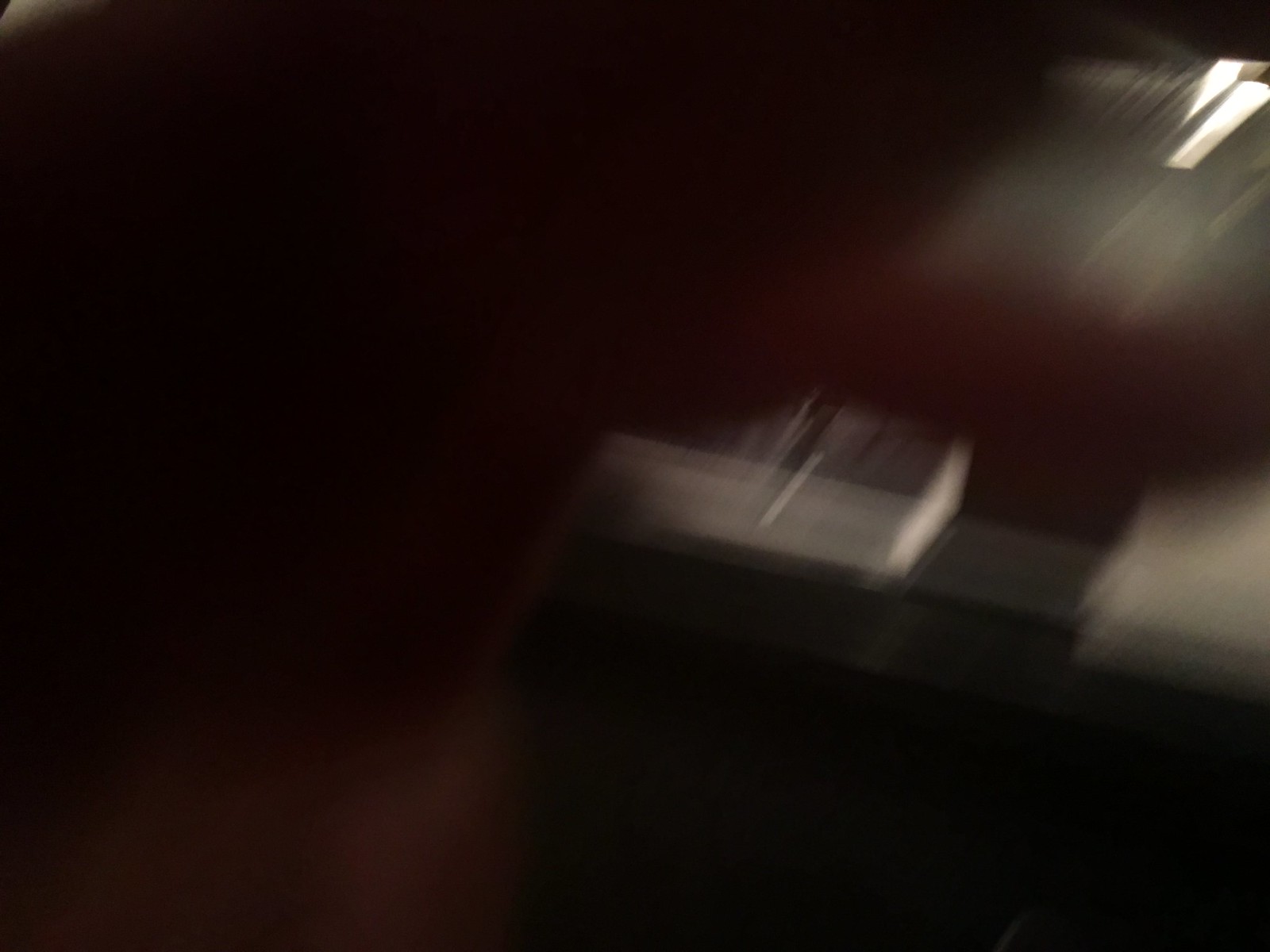This image is notably blurry and predominantly enveloped in darkness, making it challenging to discern specific details. On the lower right side, there is a black object with white appendages emanating from it, resembling either the keys of a keyboard or piano pedals positioned sideways. These white protrusions are interspersed with small gray flecks. The top right corner of the image features a bright flash or glare, indicative of light reflecting off a surface. The left half of the picture remains entirely pitch black, offering no additional details. The overall composition and poor clarity of the image add to the difficulty in identifying the exact nature of the objects depicted.